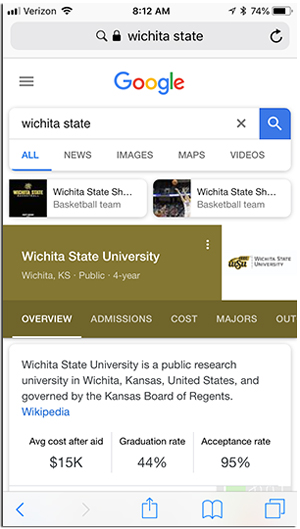On the Google search results page, the Wi-Fi signal shows full bars and the battery is at 74% with the time reading 8:12 a.m. At the top, the search bar displays "Wichita State", and immediately below it, another search bar also reads "Wichita State". 

The results are categorized under the tabs: All, News, Images, Maps, Videos, with keyword suggestions like Wichita State basketball team, Wichita State University, and Wichita, Kansas public for school, showing up under 'All'.

There's an 'Overview' tab that is bold and underlined with a white line, indicating it is selected. 

Below this, a white rectangular information box highlights the following details about Wichita State University:

"Wichita State University is a public research university in Wichita, Kansas, United States, and governed by the Kansas Board of Regents." 

The details provided are supplemented by a blue hyperlink to Wikipedia. Additionally, key statistics are listed: 

- Average cost after aid: $15K
- Graduation rate: 44%
- Acceptance rate: 95%.